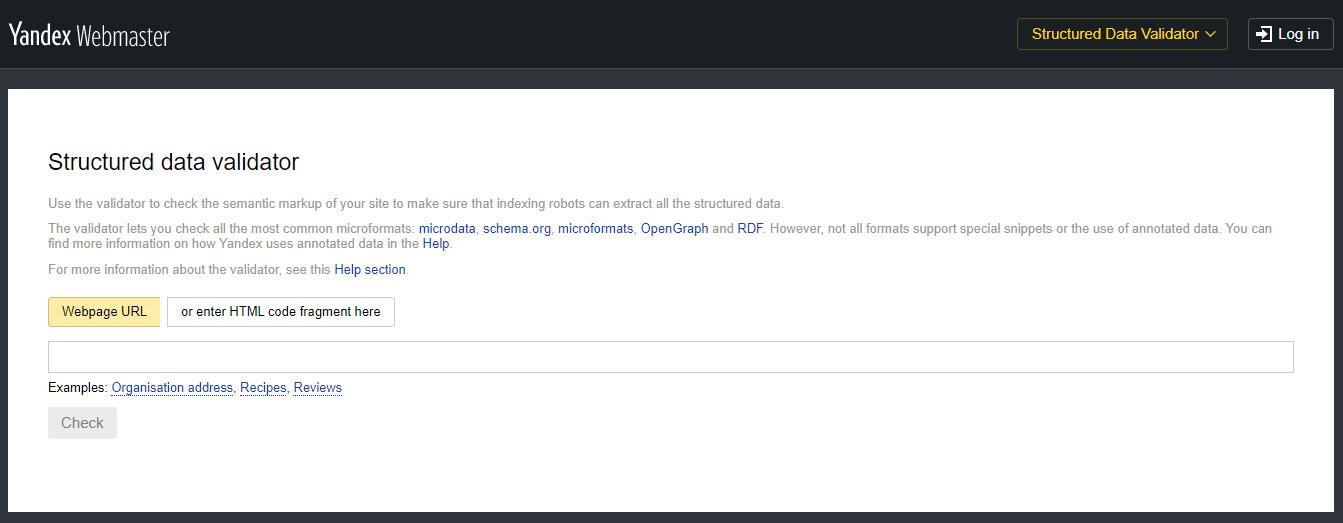This image captures the top portion of a heavily cropped website, specifically the interface of the Yandex Webmasters' Structured Data Validator. At the very top, spanning the entire width of the image, is a black horizontal bar approximately an inch thick. Below this is a lighter gray bar about a quarter inch thick.

Within the black bar, on the left side, "Yandex Webmasters" is prominently displayed in white text, with "Y-A-N-D-E-X" clearly spelled out. On the far right corner of the black bar, "Structured Data Validator" is written in yellow, accompanied by a dropdown icon to its right. Adjacent to this, there is a white box labeled "Login."

Beneath the black and gray bars, another white section reiterates "Structured Data Validator." This section contains detailed information about using the validator to check the semantic markup of websites, ensuring that indexing robots can extract all structured data properly. It enumerates the formats that can be checked and includes hyperlinks for additional help and resources.

Further down, a yellow button labeled "Webpage URL" is visible. Accompanying this, in a white box, is the text "Or Enter HTML Code Fragment Here,” followed by an input box. This input box is designed for users to enter the relevant data, and it provides example formats for reference. A "Check" button, initially grayed out, becomes active once valid data has been inputted for validation.